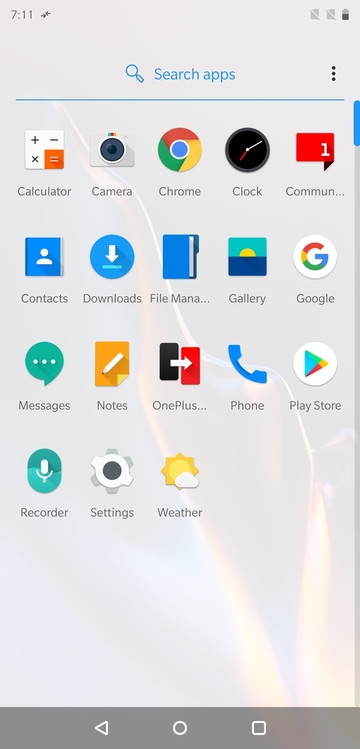Here is an enhanced and detailed caption for the image described:

"This image displays the screen of a smartphone open to the 'Search Apps' page, which is prominently located near the top of the screen. The search bar is accompanied by a magnifying glass icon, indicating where the user would input the name of the app they are searching for. Below the search bar, there are four rows of app icons. The first three rows each contain five app icons, while the fourth row has three app icons.

The specific apps displayed, from top left to right and continuing to the next row, are as follows:
1. Calculator
2. Camera
3. Chrome
4. Clock
5. Commune (partially cut off and followed by an ellipsis)
6. Contacts
7. Downloads
8. File Manager
9. Gallery
10. Google Messages
11. Notes
12. OnePlus Phone app
13. Play Store
14. Reorder (likely a feature to rearrange apps)
15. Settings
16. Weather

The background of the screen is a translucent white, allowing a faint glimpse of an image behind it. At the bottom of the screen lies a gray navigation bar containing three buttons: a back button (a left-pointing triangle), a home button (a circle), and a recent apps button (a square).

At the top of the screen, typical smartphone status icons are visible, including the time, battery indicator, and a few other notification icons."